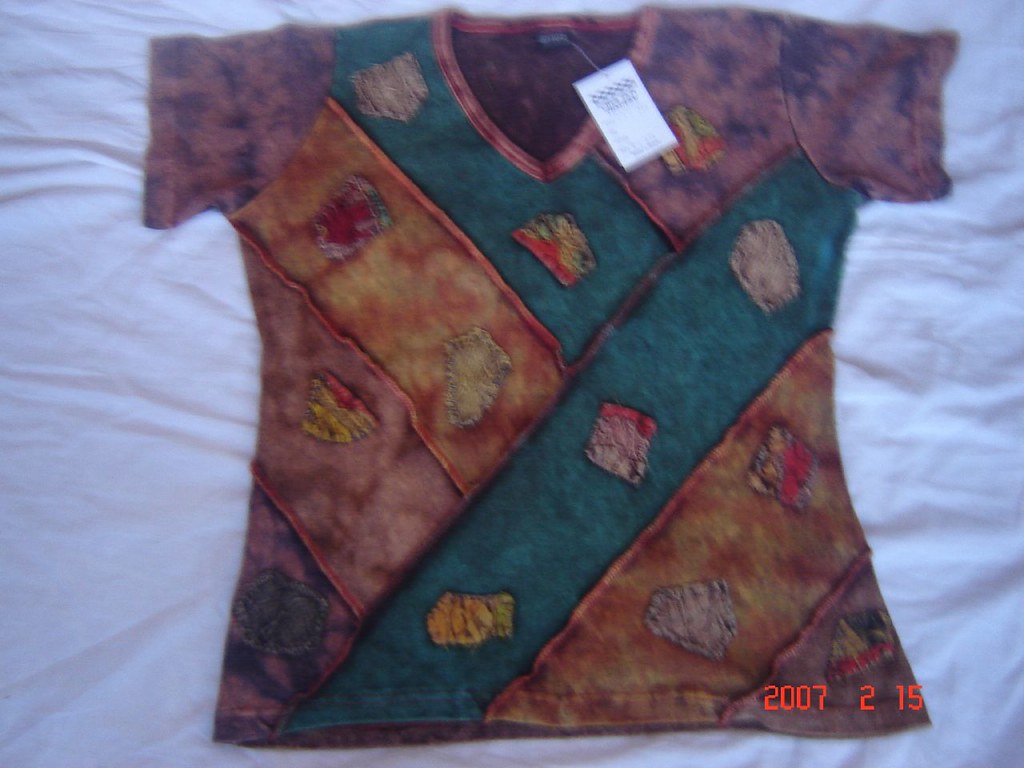This image depicts a short-sleeved, V-neck shirt laid flat on a white, wrinkled sheet. The shirt features a vibrant patchwork design with prominent colors including purple, green, yellow, and red. The center of the shirt is dominated by a large, angled green patch running from the right armpit to the bottom left, with another green patch extending from beneath the V-neck and meeting the long green strip. A yellow patch mirrors this angle, intersecting with the large green patch. Purple patches embellish both sides of the shirt, while the purple V-neck stitching and sleeves add cohesion. A white price tag with blue, blurry writing dangles from a small black tag at the back of the shirt. The bottom right corner of the photograph includes an orange digital date stamp reading "2007-2015," indicating the timeframe when the photo was taken or referencing the date in some capacity.